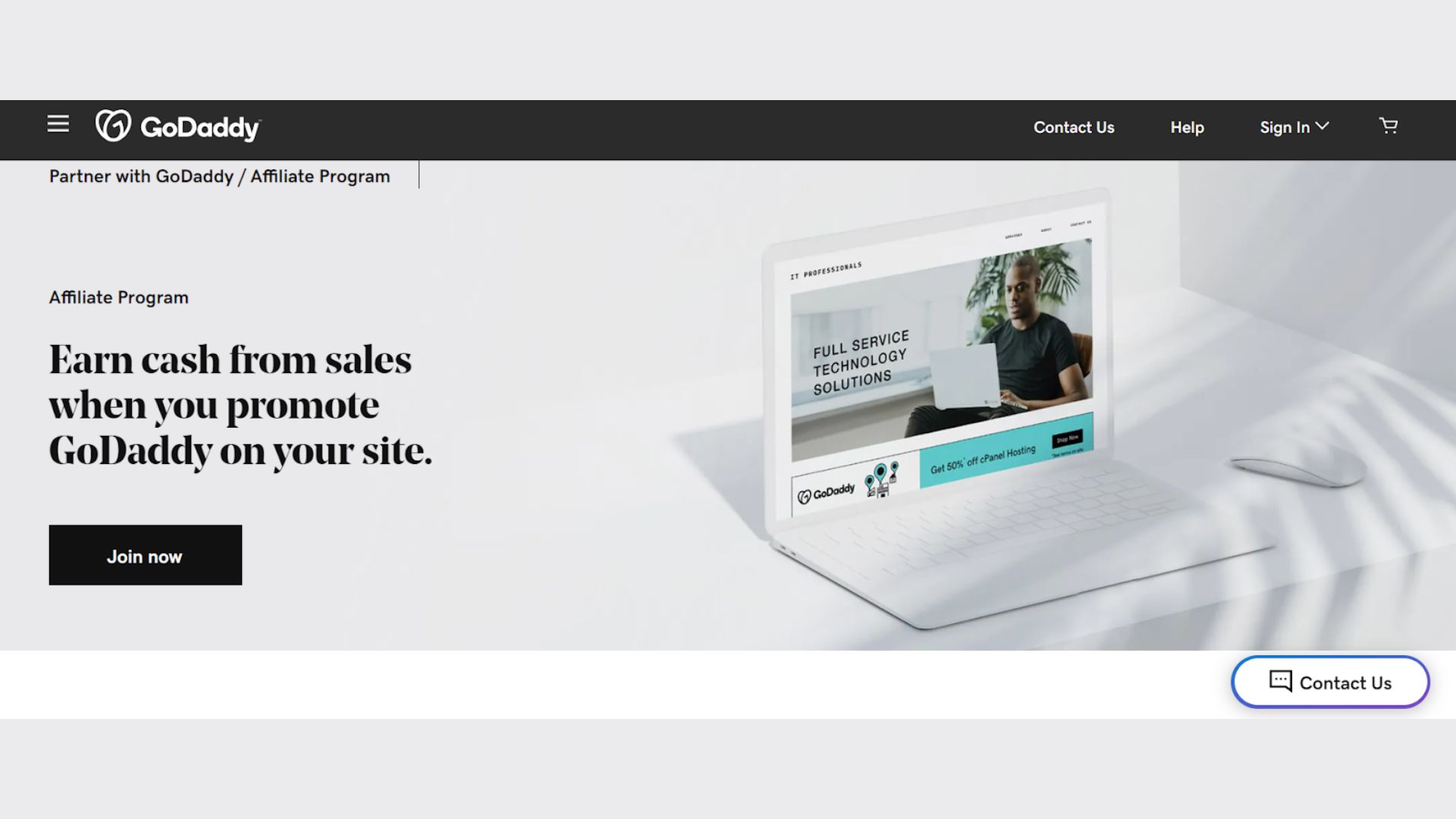**Descriptive Caption:**

In this screenshot from the GoDaddy website, the top is adorned with a black banner featuring several navigational links on the right side, namely "Contact Us," "Help," and "Sign In," alongside a drop-down menu and a shopping cart icon. Below the prominent "GoDaddy" logo, the text reads "Partner with GoDaddy / Affiliate Program." This is followed by another heading, "Affiliate Program," and a bold statement in large letters, "Earn Cash from Sales when you promote GoDaddy on your site." Adjacent to this text is a prominent black "Join Now" button.

To the right of this section, there is an image depicting a man comfortably seated in an easy chair with a laptop on his lap, actively typing on the keyboard. This image is accompanied by the caption, "Full Service Technology Solutions."

At the bottom left of the screenshot, the "GoDaddy" logo is displayed once more. Accompanying it is a somewhat blurred blue banner with illegible text. On the bottom right is another "Contact Us" note, paired with a button and a blue bar, devoid of any pictures or text. The entire screenshot predominantly features a light blue color scheme, offset by black text and the central image of the man with the laptop.